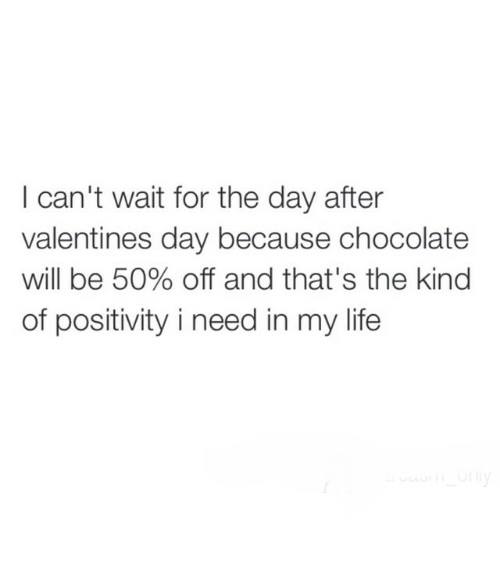The image features a simple design with a completely white background and no borders, allowing a significant amount of blank, empty space. Positioned centrally in the image, black text spans four lines: "I can't wait for the day after Valentine's Day because chocolate will be 50% off and that's the kind of positivity I need in my life." There are no other visual elements or colors, making the focus solely on the text, which delivers a satirical, humorous message suitable for social media sharing. Notably, the word "I" in the phrase "positivity I need in my life" is in lowercase, contrasting with the capitalization at the beginning of the sentence.